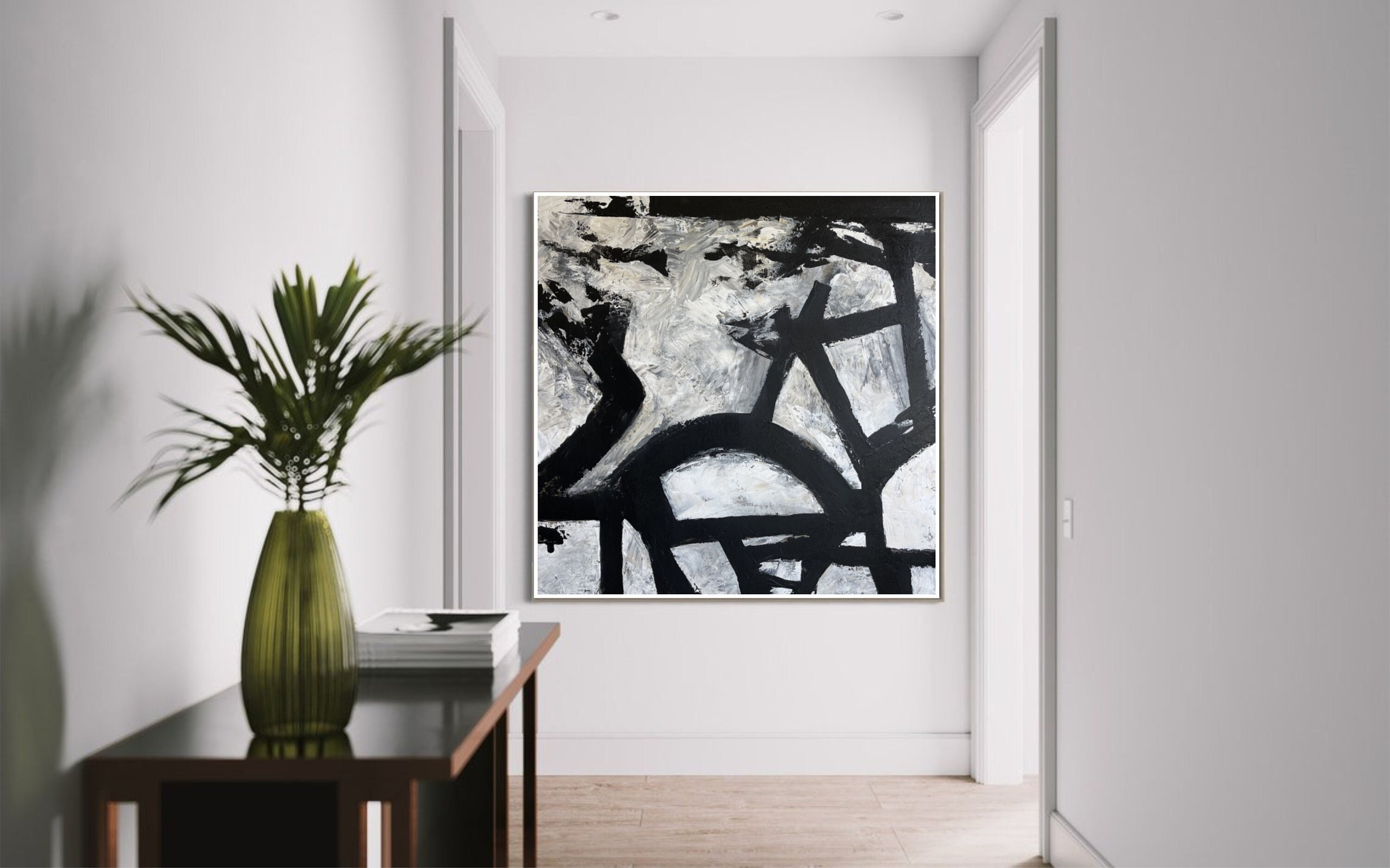The image depicts a narrow, indoor hallway with white walls and a light brown wooden floor. At the end of the hallway, there is an abstract painting mounted on the wall. The painting features a white background adorned with black shapes, including a half-circle, zigzag lines, and a square-like angle. Adjacent to this back wall are two doorways: the one on the right emits bright light, likely from a window or an open door, while the left doorway appears dim. A small, dark brown wooden table is situated against the left wall of the hallway. Atop the table, closer to the front, stands a tall, thin green vase with palm fronds sprouting from it, and towards the back, there is a stack of white papers or magazines.